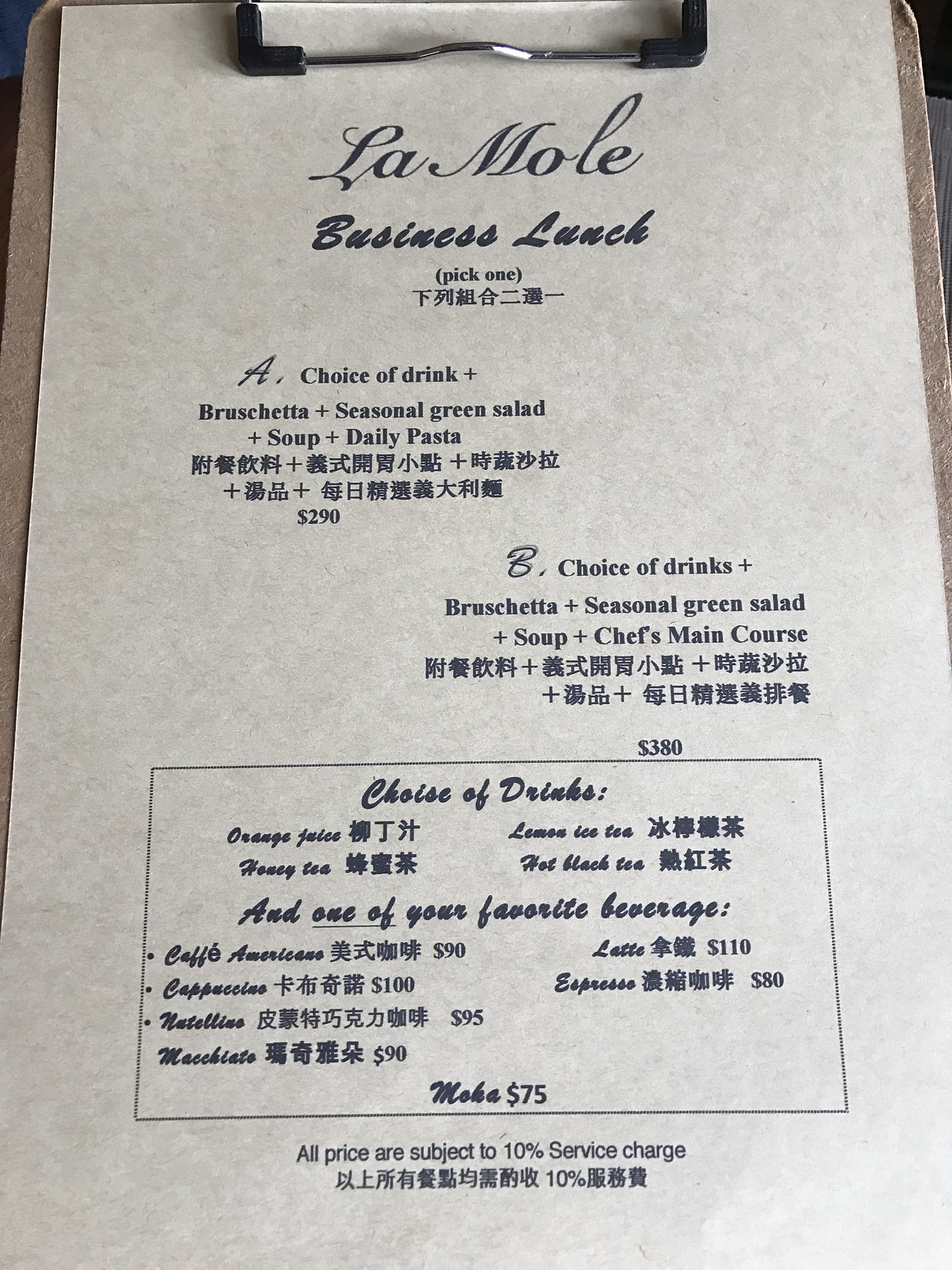The image features a color photograph of a menu clipped to a particle board clipboard. The menu is the sole focus of the image. At the top center, the restaurant's name is displayed prominently: "L.A. M.O.L.E." Below the restaurant name, the heading "Business Lunch" introduces the menu options available.

The menu offers two main choices for lunch, labeled as Choice A and Choice B. 
- **Choice A** includes Bruschetta, a Green Salad, a Soup, and the Daily Pasta, priced at $2.90.
- **Choice B** consists of Bruschetta, a Green Salad, a Soup, and a Main Course, priced at $3.80.

Both choices are accompanied by Chinese characters, providing translations for non-English-speaking patrons. 

The bottom third of the menu is bordered and lists various drink options, including coffees and teas. At the very bottom, there is a note indicating a 10% service charge, also represented in Chinese characters.

The menu itself appears to be printed on heavy cardstock, clipped neatly to the clipboard, ensuring it is readily accessible for the server's use.